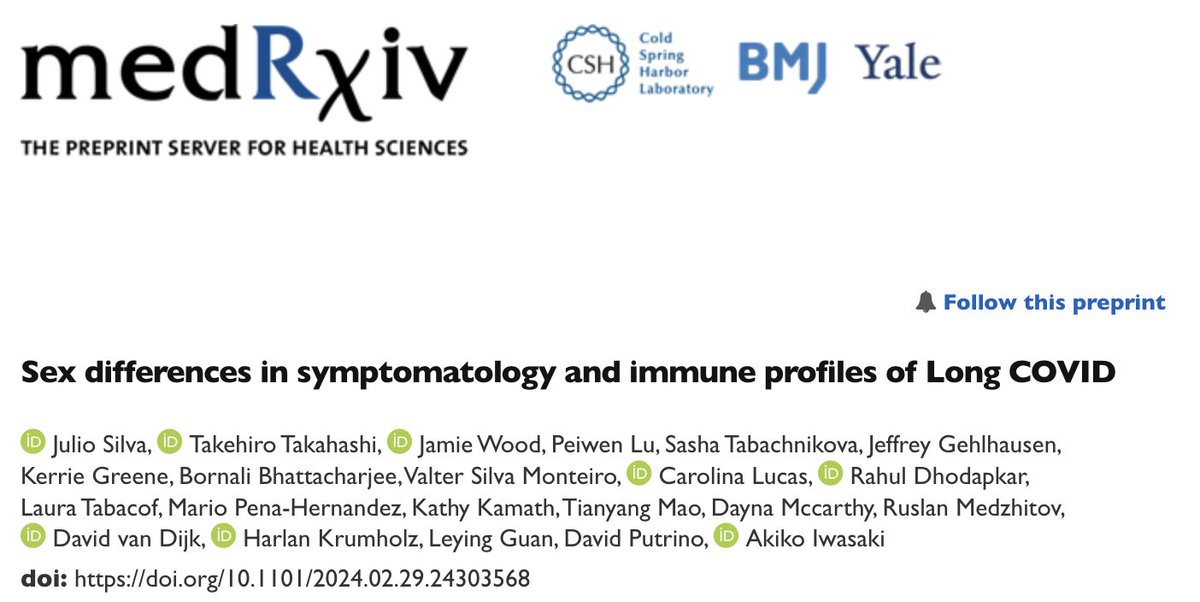This image, set against a white background, contains various text elements and icons arranged in a structured layout. 

In the upper left corner, the text "medRxiv" is prominently displayed. The letters "med" are in large, black lowercase font, the "R" is in capital blue, while the "X" extends slightly below the baseline. Following this, "IV" is in black. 

To the right, a logo is visible, and next to it, aligned vertically and in blue font, are the words: 

- "Cold"
- "Spring"
- "Harbor"
- "Laboratory"

Continuing further to the right, "BMJ" is written in blue uppercase letters, and adjacent to it, "Yale" is in black.

Moving back to the left side, approximately three lines below, a bold and all-caps inscription reads, "THE PREPRINT SERVER FOR HEALTH SCIENCES." 

About seven lines down on the right edge, there is a black bell icon followed by blue text stating, "Follow this preprint." 

Approximately three lines down, another bolded black text reads, "SEX DIFFERENCES IN SYMPTOMOLOGY AND IMMUNE PROFILES OF LONG COVID."

After about two blank lines, there is a green circle resembling a light with a white capital "ID" inside it. To the right are names separated by commas and preceded by the green circle, which repeats for four rows.

Then there is a blank row, followed by the text "doi:" in bolded black lowercase, succeeded by a specific website address.